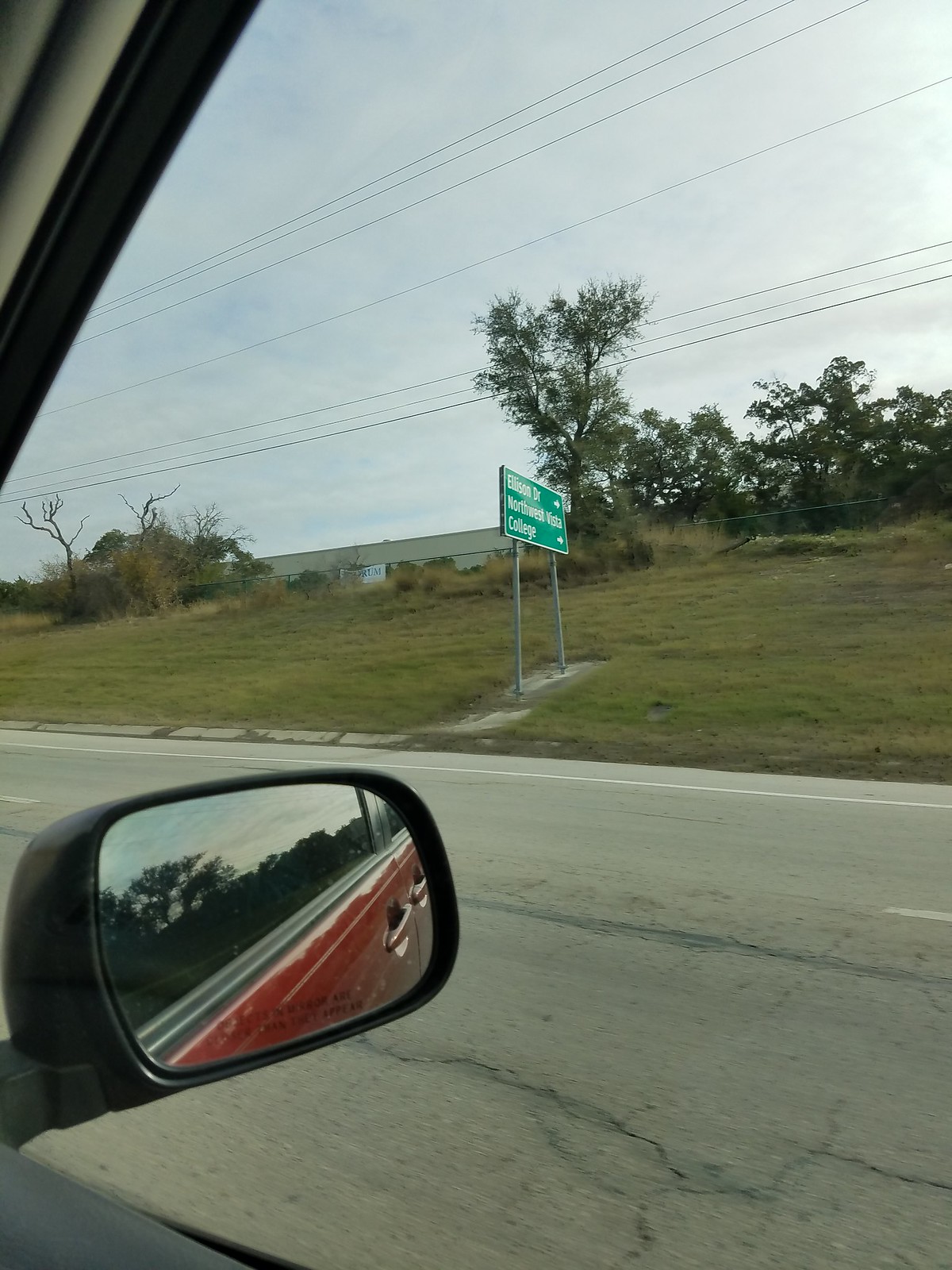This vertical color photograph captures an evening view from inside a burgundy car, looking outward through the passenger window. Dominating the scene is a large green road sign mounted on two silver poles, positioned on an unkempt grassy hillside that appears to run alongside a highway. The sign, which reads "Ellison Drive" and "Northwest Vista College," features two white right-pointing arrows. The reflection in the car's side mirror, depicting the red body of the car, is clearly visible on the left of the image.

In the background, a diverse array of trees, some appearing tall and lush while others are bare and possibly dead, are scattered across the hill. These are accompanied by an overgrown bush on the left and additional clusters of trees on the right. A partly cloudy sky, rendered in light gray tones with hints of blue, forms the backdrop, intersected by telephone and electric lines that run horizontally across the image. Only the upper portion of a building, peeking over the hill, is visible in the distance. The road in the foreground is slightly cracked and runs parallel to a chain-link fence with a white banner on it. The overall ambience reflects an overcast evening with elements of nature and urban infrastructure blending seamlessly.